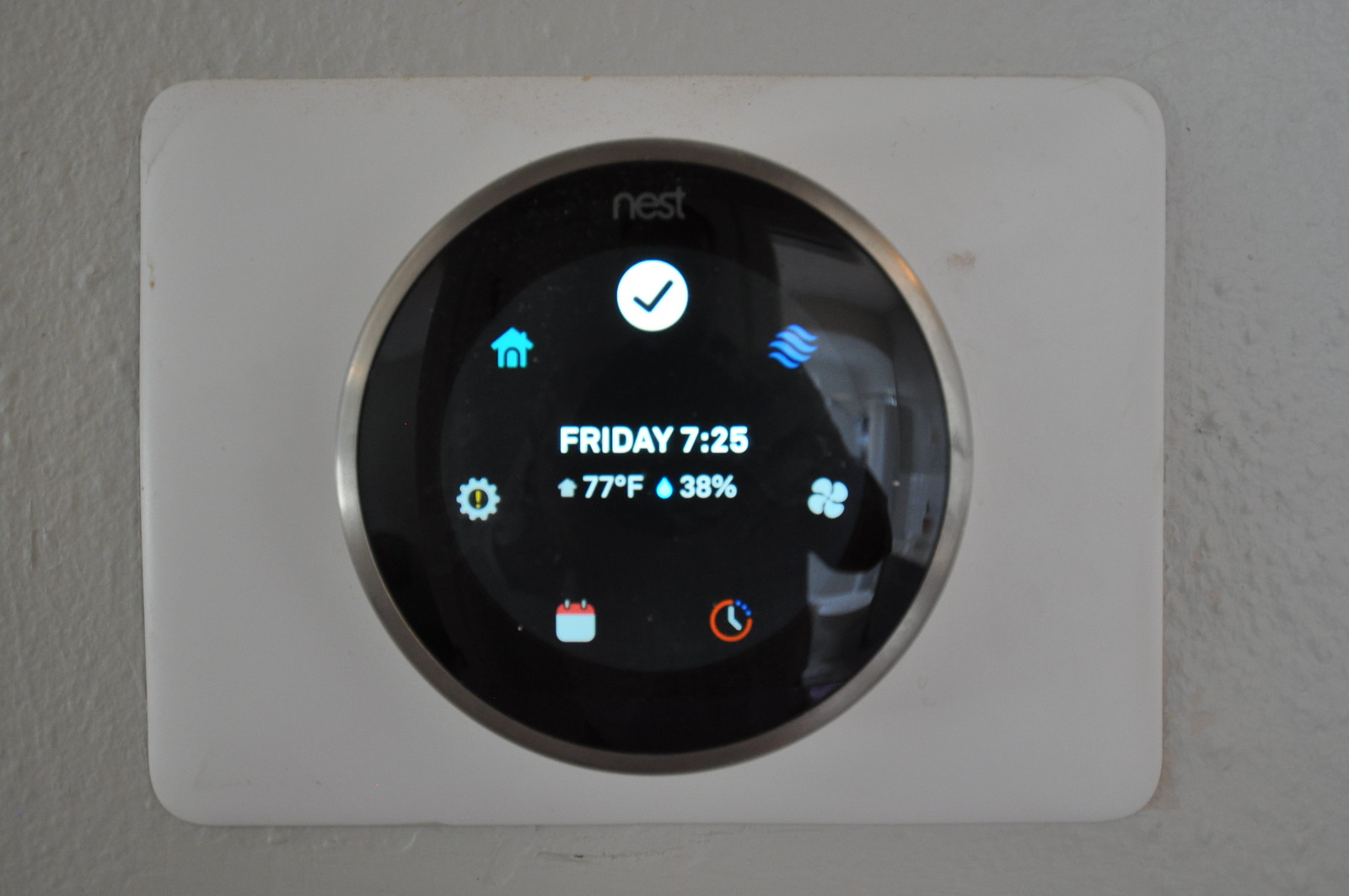The image captures a sleek, modern thermostat known as a Nest, mounted on a textured white wall. The thermostat is a white rectangular device featuring a prominent silver circular interface. At the center of this circle is a black display screen. Prominently, the word "Nest" is inscribed on the upper section of the device.

The display screen provides detailed information, highlighting it’s Friday at 7:25. An icon of a house is shown, alongside the current temperature of 77 degrees Fahrenheit. Below these details, there is a water droplet icon indicating the humidity level at 38%.

Encircling the display are seven distinct icons arrayed around the silver bezel. At the 12 o'clock position, there is a checkmark symbol. Moving clockwise, the next icon at about the 1:30 position comprises four blue swirls, likely representing airflow. The 4 o'clock position features an icon of fan blades. Positioned at around 5:30, a timer or clock symbol is shown with an orange three-quarter circle and hashed blue quarter circle. At the 7 o'clock position, there is a calendar icon. Around 9 o'clock, a gear symbol is displayed with a yellow exclamation mark inside it. Finally, located in the upper left quadrant, near 10:30, there is an icon of a blue house.

The image presents a comprehensive and detailed view of the Nest thermostat, showcasing its modern design and functional interface.